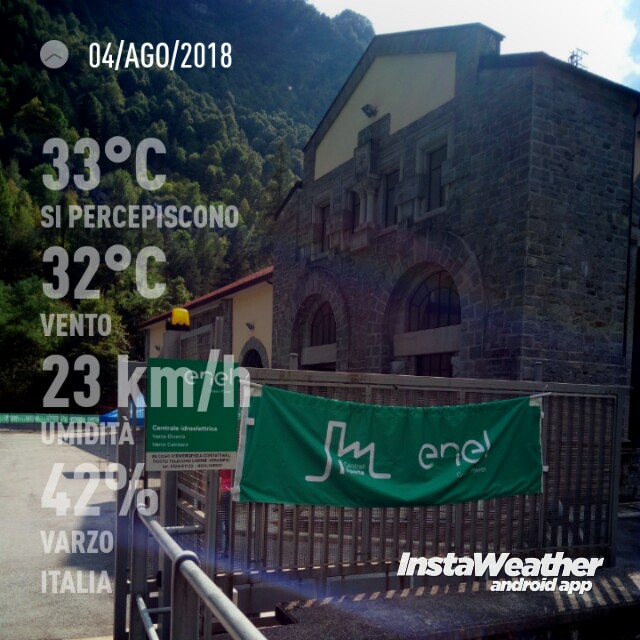This somewhat faded, full-color photograph, taken outdoors on a somewhat sunny day, appears to be a screenshot from the InstaWeather Android app. It displays a date of 4th of August 2018 and various weather details, indicating a temperature of 33 degrees Celsius, wind speed of 23 kilometers per hour, and 42% humidity. The text, primarily in Italian, includes the word "Italia" at the bottom. The scene features a metal fence or guardrail adorned with a green flag bearing white print, positioned near an old missionary-style building made of dark gray stone, which is situated at the foot of green trees. The left side of the image shows small mountains in the background. The app's logo, which is in a bold, italicized sans serif font, is prominently displayed in the bottom right corner.